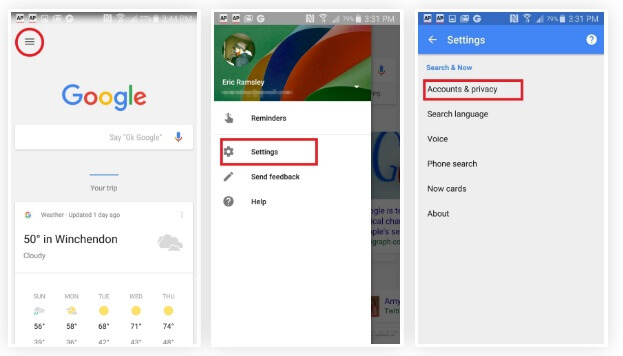This image, captured on an iPhone, spans three distinct pages. 

**First Page:**
The screen is predominantly light-colored with a faint visibility of the battery life indicators at the top, appearing grayed out. Central to this screen is a large, prominently displayed word "Google" featuring its characteristic blue, red, gold, and green colors. Below this title is a white search bar with the text "Say 'OK Google'" and an adjacent microphone icon. Encircled in red are three horizontal lines, drawing attention to a menu option. Below the search bar, a small blue banner provides weather update details where "Your Trip" information is highlighted with a weather status indicating it was last updated a day ago. It shows a temperature of 50 degrees with conditions labeled as cloudy. An icon of a cloud is present alongside a weekly forecast spanning from Sunday to Thursday, detailing the high and low temperatures and whether it will be sunny or cloudy for each day.

**Second Page:**
This page features what appears to be the profile of someone named Eric Ramsley. His profile image is displayed in a circular frame adorned with colors resembling a large hot air balloon: red, blue, and yellow. Below his image, the interface includes options such as "Reminders", highlighted with a toggle feature, and a settings button enclosed in a red box. Additional options on this page include "Send Feedback" and "Help".

**Third Page:**
Set against a blue backdrop, this screen provides various settings options. More of the phone's icons along the top edge are visible here. Main headings include "Search & Now", "Accounts & Privacy" (outlined in red), "Search Language", "Voice", "Phone Search", "Now Cards", and "About". Most of these options appear in a gray font, indicating subsections and additional functionalities.

This comprehensive description captures the intricate details presented across the three screens, offering a vivid portrayal of the content displayed on the iPhone.